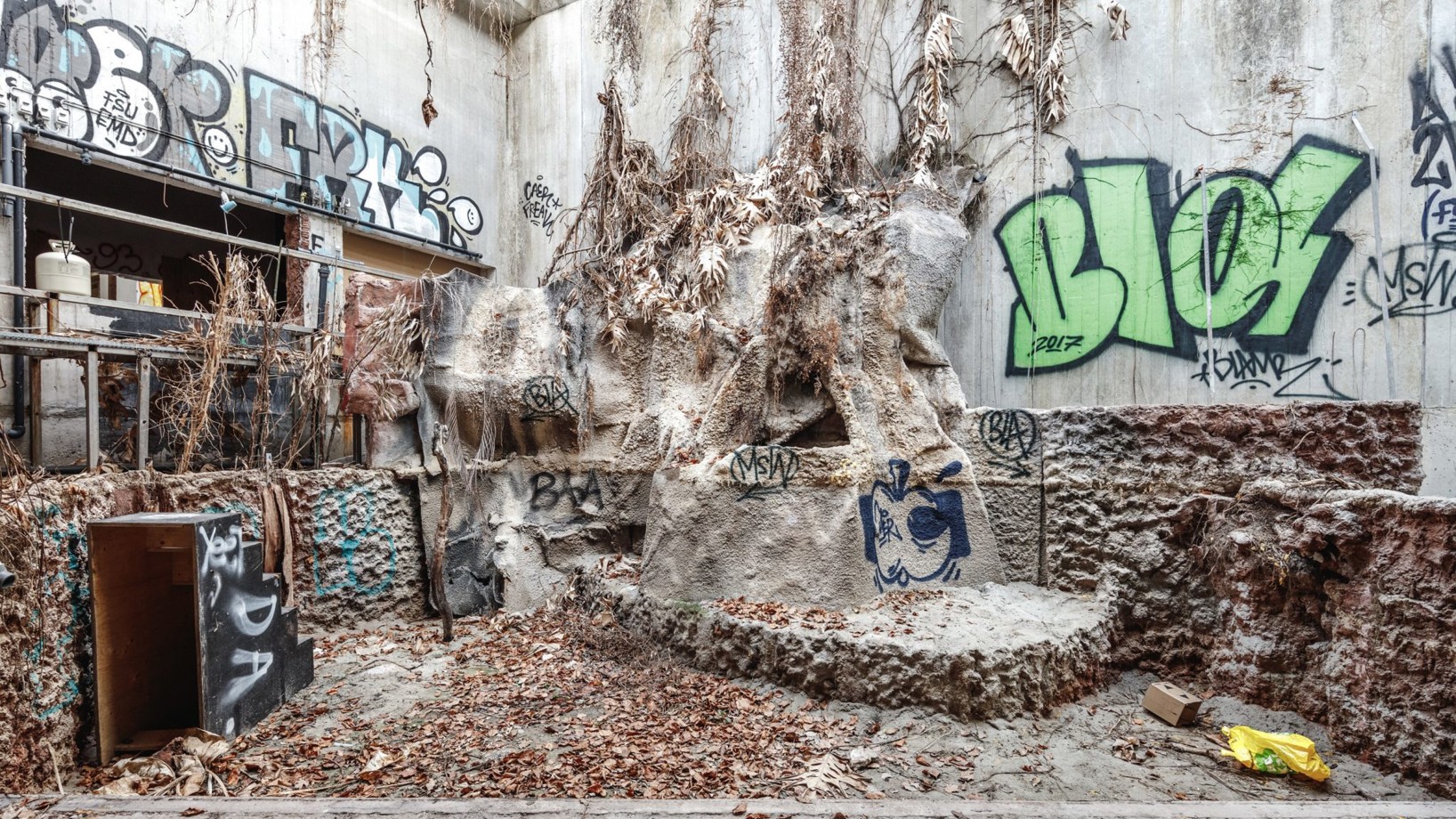The photograph depicts a dilapidated, possibly abandoned, outdoor corner area surrounded by concrete walls. The ground is strewn with dirt, dead leaves, and remnants of dead plants, some of which climb the walls like skeletal branches. The scene is illuminated by natural daylight, suggesting that a part of the roof may have collapsed, flooding the area with light. 

The graffiti is prominent and varied: on the bottom left, a black movable staircase has "D and A" scribbled in white. Towards the center-right, "BIOS" is written in green, surrounded by indistinct black scrawls. On the top left, there's a difficult-to-decipher, stylized gray and white graffiti featuring letters like R, F, and K. Additionally, another piece is visible in green on the right wall, potentially reading "BLOK" or "BIOS," with black marks that suggest further graffiti, including a possible artist's signature and the year 2017 inscribed. The overall scene has an air of decay and neglect, with broken window frames and an array of discarded objects scattered around, hinting at the possibility that this space might have once been part of a larger structure, such as a shopping mall or an alleyway between buildings.